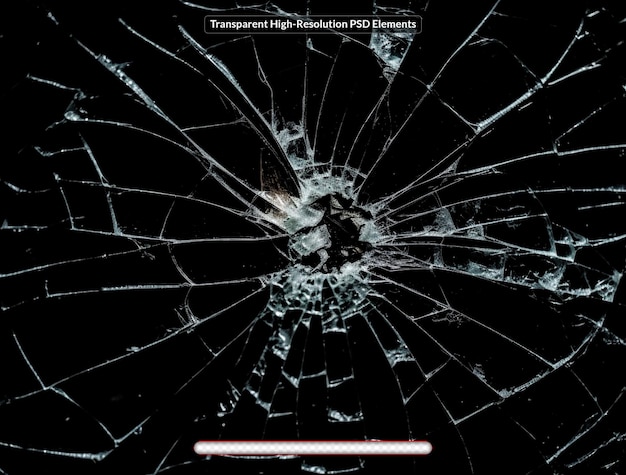This image is a high-resolution photograph with a pitch-black background, featuring a shattered glass or windshield in the center. The top edge of the image is marked by the white text: "transparent high-resolution PSD elements." The shattering converges on a central point where a large, jagged hole is surrounded by numerous smaller shards, resembling a spiderweb pattern. Radiating from this center are white streak-like cracks of varying widths and lengths. The image suggests that an impactful force, possibly a bullet or similar object, caused the damage. A thin white line or fluorescent strip is visible at the bottom edge of the image, the purpose of which remains unclear. The detailed pattern of the cracks and shards hints that even the slightest further pressure could cause the glass to break into fragments.